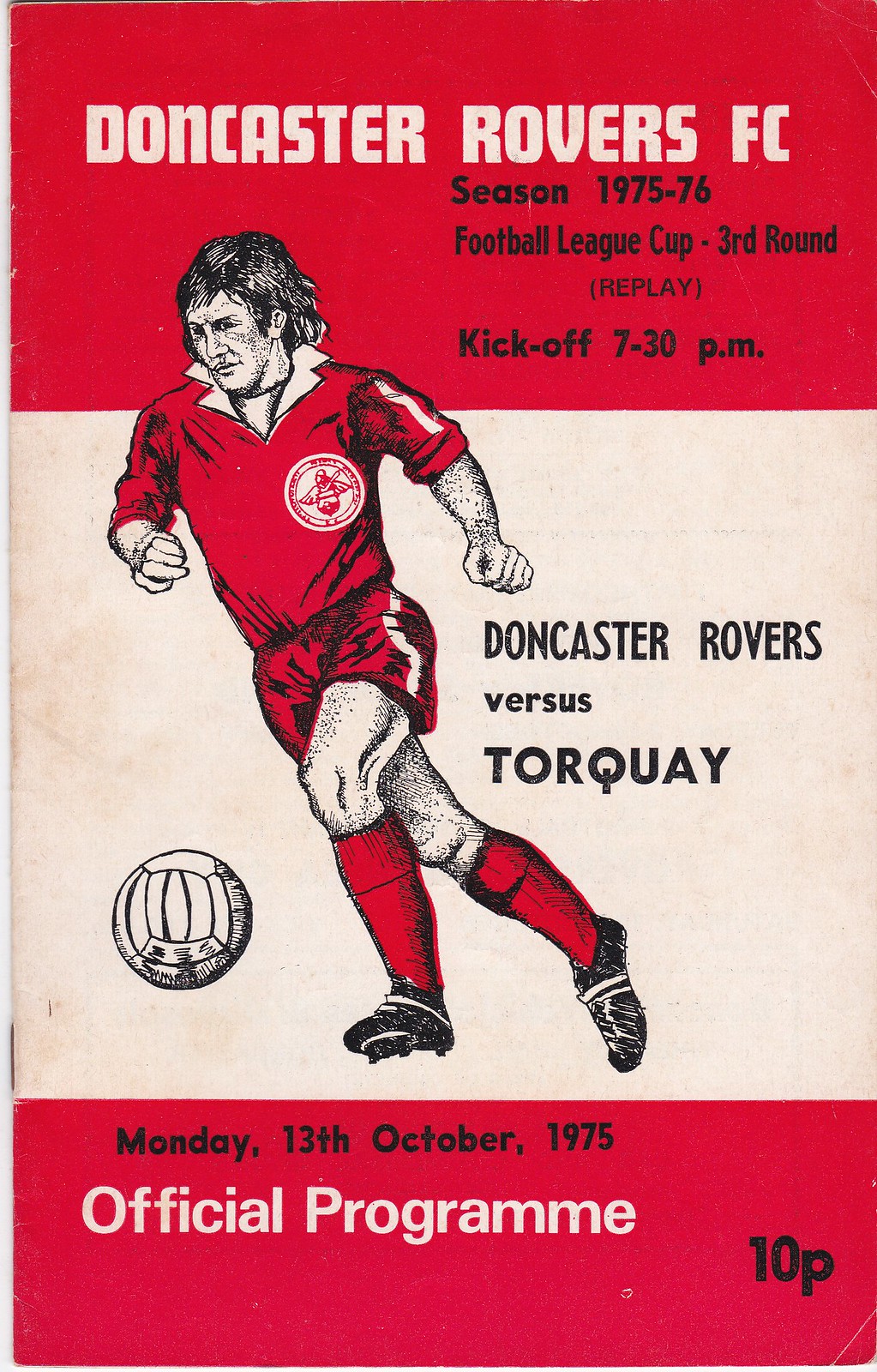The image is the official program cover from the Doncaster Rovers FC for the 1975-1976 season, specifically for the Football League Cup 3rd Round replay match against Torquay, held on Monday, October 13th, 1975, with a kickoff at 7.30pm. The cover, priced at 10 pence, features a detailed drawing of a soccer player with dark brown hair, dressed in the red uniform of Doncaster Rovers FC, preparing to kick a ball. The design is predominantly red with black and white text, and includes a white and red logo on the player's shirt. The image emphasizes the absence of advertisements, focusing solely on the player and the event details, ensuring a clean and visually striking presentation. The word "replay" is notably placed within round brackets.